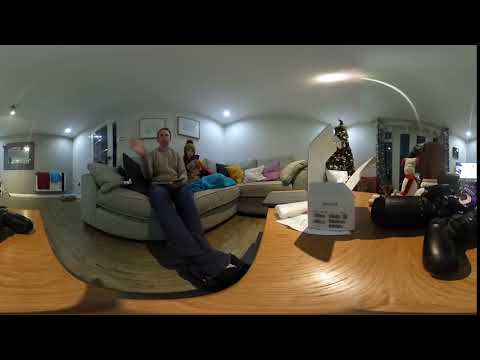In an image depicting a cozy living room, a man and a young girl are seated on a tan-colored sofa, surrounded by an array of vibrant pillows in shades of pink, yellow, white, blue, and tan. The man, dressed in a tan shirt and blue jeans, appears to be waving, while the young girl beside him wears a winter hat. His legs appear disproportionately long, likely a result of distortion from the wide-angle camera used, which has given the photograph a somewhat curved, panoramic effect. The sofa is draped with a blue blanket, and a stuffed animal with a red ribbon is also visible. 

Behind them, a decorated Christmas tree adorned with clear lights stands against a backdrop of white walls, with additional blue and white striped wallpaper to the right of the tree. The room is lit by ceiling can lights and additional lights positioned in the corners. A wooden desk or table can be seen in the foreground, further emphasizing the curve of the wide-angle lens. Various picture frames, including a mirror with a gray frame, embellish the walls, enhancing the homely atmosphere. The hardwood floor's dark and light brown tones add warmth to the scene. This indoor snapshot, likely taken in someone's living room, visually encapsulates a festive, intimate family moment.